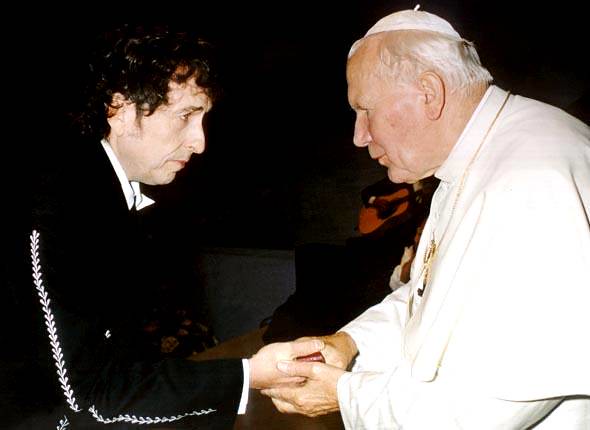In this photograph, a person resembling Bob Dylan is meeting the Pope. The individual on the left, who appears to be Bob Dylan, has a right profile showing his medium-length curly brown hair. He is attired in a black long-sleeve sweater or jacket that features decorative lines down the sleeves, along with a white shirt underneath. He extends his right hand to the Pope. The Pope is visible on the right, facing left, wearing a traditional white robe and a rounded white cap. His profile reveals his white hair, and he holds Bob Dylan’s hand in both of his hands, with a hint of golden adornment visible on the front of his outfit. The background of the image is predominantly dark, revealing only a light-colored wall in the middle and a guitar beneath the Pope's chin, suggesting someone is playing it.